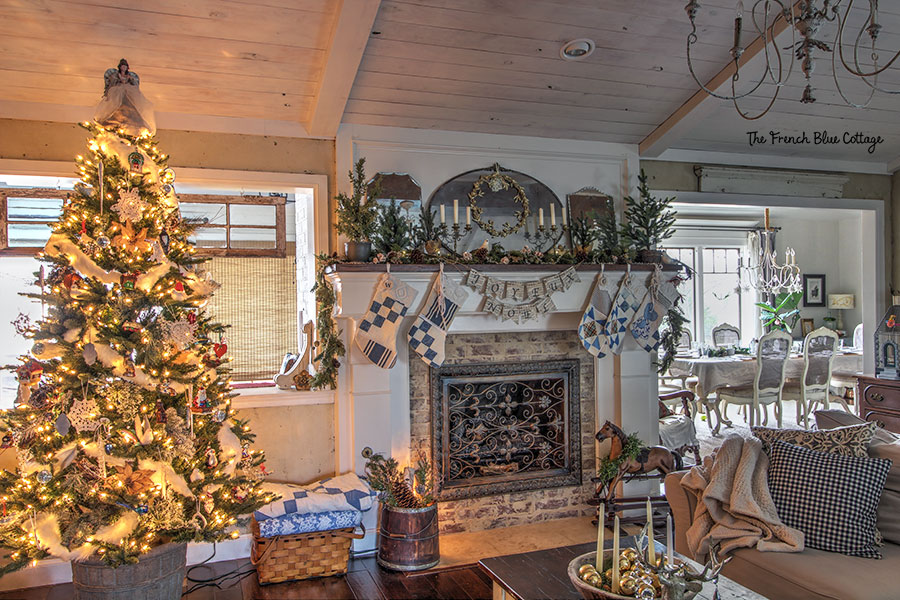Inside the French Blue Cottage, this horizontally aligned rectangular image captures a cozy and festive atmosphere. The slanted wooden ceiling, painted white, features spotlights and the cottage's name artfully written in the upper right corner above a doorway leading into a dining room. The dining room showcases a table draped in a white tablecloth, surrounded by tall-backed white wooden chairs, and adorned with plates and place settings.

In the lower right corner of the picture, you can see the end of a sofa accented with a black and white checked throw pillow and a cozy blanket. Adjacent to the sofa, a coffee table is decorated with a variety of knick-knacks and candles. Dominating the center of the room, a fireplace is framed by gray and white bricks and ornate gold bars. Stockings are hung across the mantle, with the word "Joyful" visible among the decor. A mirror and additional decorations, including candelabras, sit atop the mantle.

To the left of the fireplace, a Christmas tree stands festooned with white ribbons and crowned with an angel topper. Behind the tree, light filters through curtains that are a delicate beige. Completing this homely scene, a small rocking horse rests in front of the fireplace, adding a touch of nostalgic charm. The overall aesthetic is warm, inviting and holiday-ready.